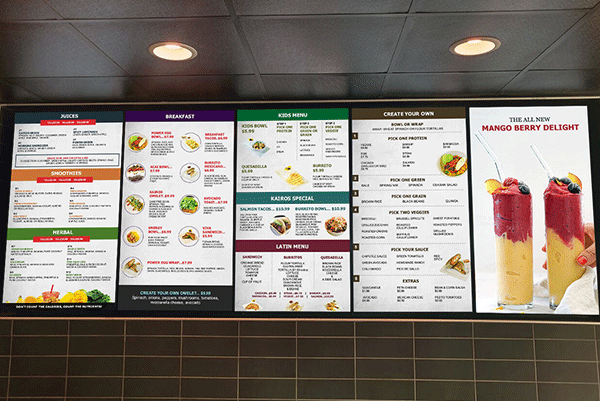In this detailed photograph of a fast food restaurant's illuminated menu board, mounted against a distinctive brown tile wall with gold lines, the entire menu is clearly visible. The wall features a striking appearance of gold lines and a black ceiling, accented by two strategically placed bucket lights illuminating the menu from above. 

The menu comprises five distinct sections, each on separate boards. Starting from the left, the first board is divided into three categories: at the top are various drinks, including smoothies and herbal drinks. The middle board highlights breakfast options with vibrant, appealing images. Moving right, the next section showcases the kids' menu, daily specials, and a Latin menu, all accompanied by colorful pictures of the food items on offer. The fourth section invites patrons to create their own menu items, providing a customizable dining experience. 

Lastly, the far-right board prominently features the all-new mango berry shakes, depicted in tall glasses adorned with fruit slices and straws. The shakes appear with a bottom layer of mango and a top layer of a raspberry-colored blend. Overall, the menu emphasizes a variety of healthy food choices including tacos, burgers, salads, and numerous side dishes, well-suited for health-conscious patrons. The white background of the menu boards contrasts effectively, making the images and text easily readable for anyone standing at the counter.